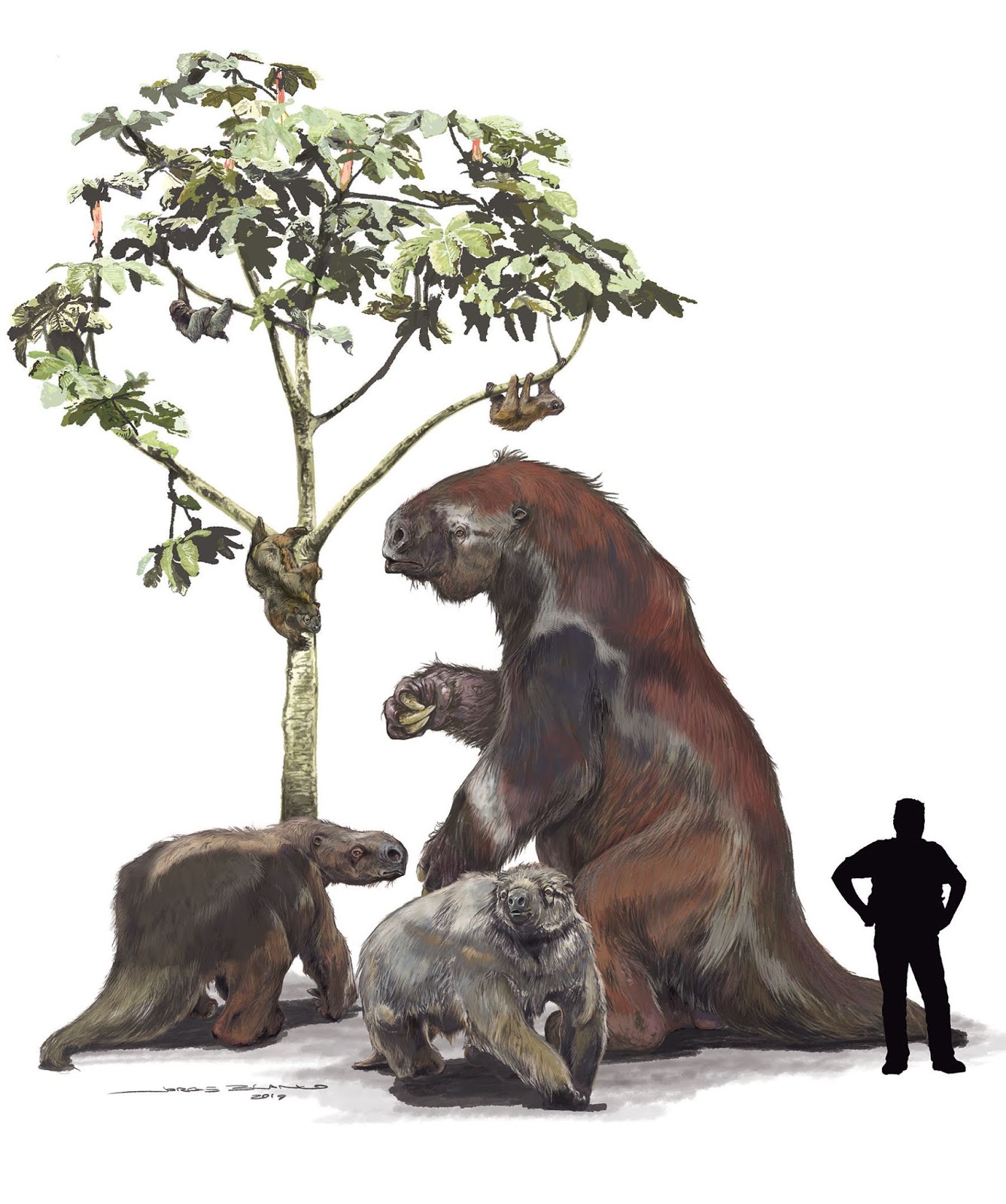The image is a detailed painting depicting an intriguing comparison between prehistoric giant sloths and an average-sized human. On the right side, there is a small black silhouette of a man standing with his hands on his hips, emphasizing the scale of the creatures. The background is white, enhancing the contrast between the figures and the environment.

On the left half, there's a tall tree with a foliage top, home to three smaller sloths hanging from its branches. These sloths appear to be of a size comparable to modern sloths. Beneath the tree, the ground hosts three much larger sloth-like creatures, presumably ancient giant sloths. Two of these giant sloths are standing on all fours near the base of the tree, their heads aligned with the mid-height of the tree. The third and largest sloth sits upright, facing left, towering at twice the height of the human silhouette.

The sloths exhibit shades of gray and brown and are rendered in a detailed yet non-photorealistic style. The artist’s signature in the bottom left corner, dated 2019, confirms it as a contemporary interpretation of these prehistoric creatures. Overall, the painting vividly contrasts the immense size of ancient sloths with modern humans and their more common descendants, all set against the striking simplicity of the composition’s white background.